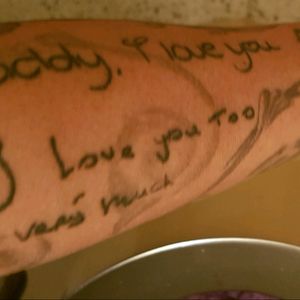The image is a close-up of a light-skinned man's forearm resting over a bowl of dog food. The arm features black ink handwriting in a child's script, which reads, "Daddy, I love you," followed by "Love you too." Beneath these lines, some additional, less legible writing is visible, accompanied by swirls of gray. The arm also has a visible tattoo underneath the handwritten messages. The background features a white table with a cream-colored backdrop, and part of the man's shirt is visible on the left side of the picture. The bottom right corner shows a concave metal object, possibly part of the bowl.